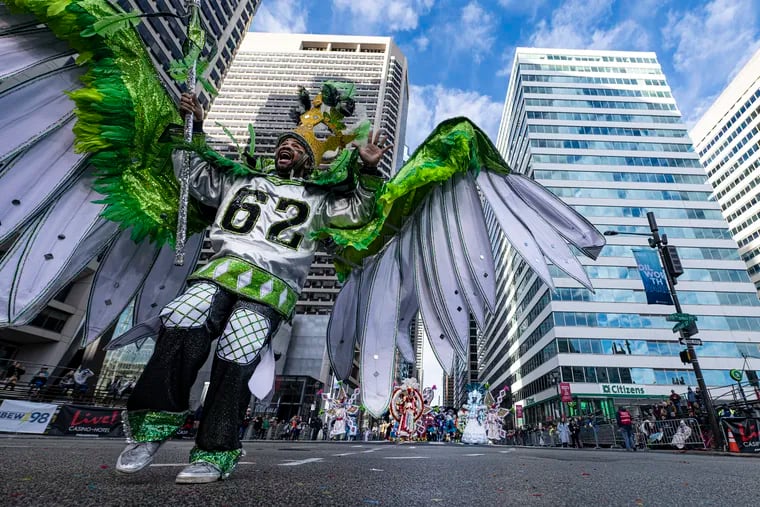The image captures a lively parade on a sunny day, with barriers and crowds of spectators lining both sides of an asphalt street. At the forefront stands a man in a festive green and white costume featuring a white sports jersey with the number 62 outlined in green. He wears black pants adorned with mesh detailing on the front thighs and green-patterned hems, along with white shoes. His elaborate headdress is a large gold crown, embellished with green elements sticking out from the top, and he has his arms raised, mouth open as if yelling or chanting, exuding joy and energy. Behind him, the backdrop is bustling with more costumed participants, juxtaposed against tall office buildings, one notably marked with a Citizens Bank logo. The clear blue sky and scattered clouds complete this vibrant scene, suggestive of a Mardi Gras celebration.